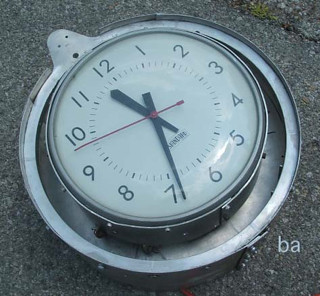This image features a clock lying on its back on the ground, with its top frame removed. The clock appears to be nestled inside the back side of its original frame, resembling a shallow bowl. The clock face is white with black numerals. The clock is positioned at an angle such that the numeral six is directed towards the lower right corner of the image. Additionally, the letters "BA" are visible in the lower right corner, seemingly added to the image post-production.